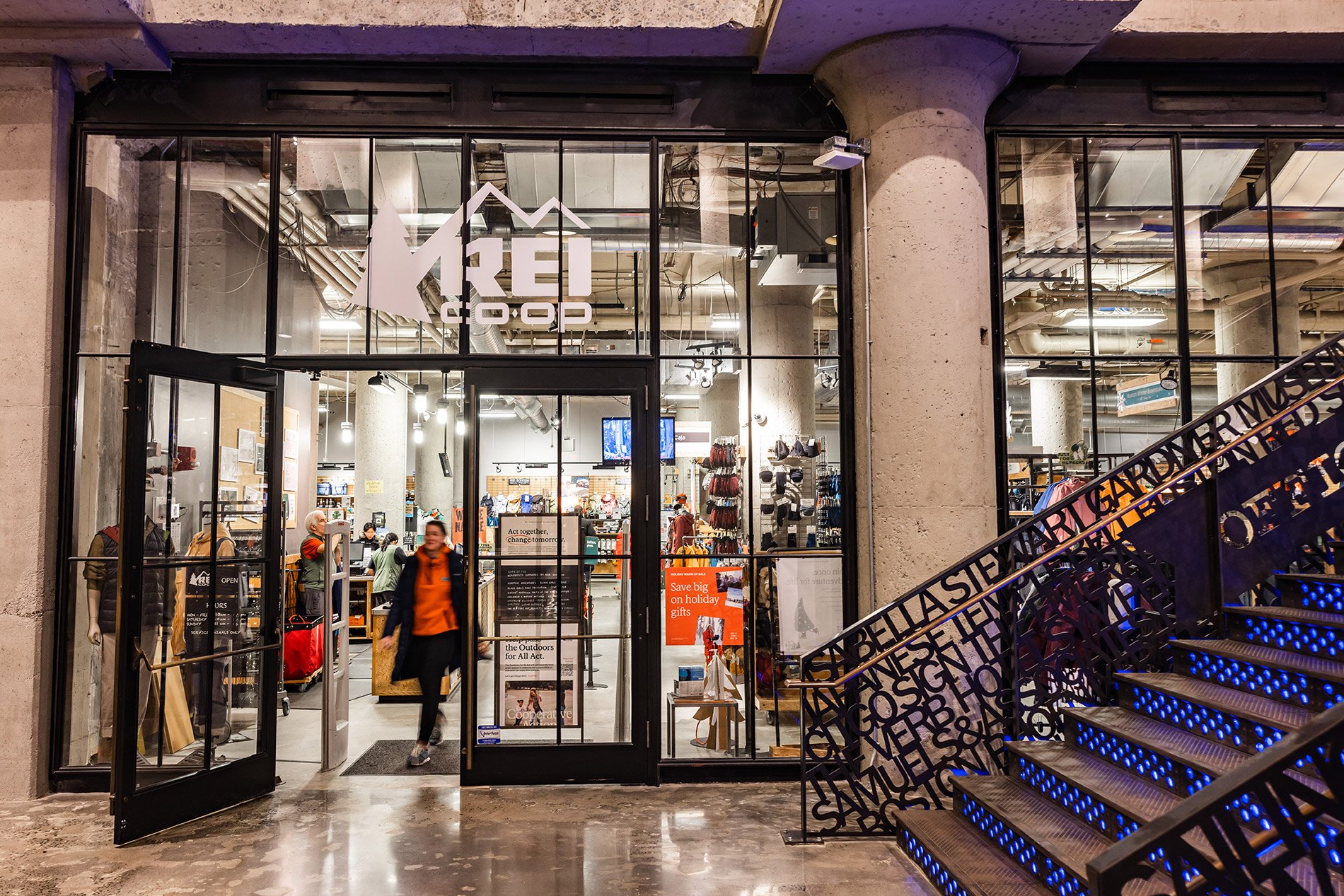This photograph captures the storefront of an REI Co-op store located inside a mall. The store features a glass facade with black trim between the large glass panes and a prominent stone pillar near the entrance. Above the glass double doors, which have a black frame, the REI Co-op logo is displayed in large white letters along with a mountain design and a pine tree. There is a tan marble floor and a staircase with illuminated blue lights on each step, accompanied by a metal railing adorned with various words and names.

A woman is walking out of the store, wearing a black jacket over an orange fleece, with black pants. She is passing through the wide-open door and the metal detector area. Inside the store, racks of clothing, a couple of employees, and a cashier working at the register area are visible. A TV screen is mounted on the far wall, and the ceiling is well-lit. The overall ambiance suggests an upscale retail environment with neatly displayed merchandise including clothing, shoes, and accessories.